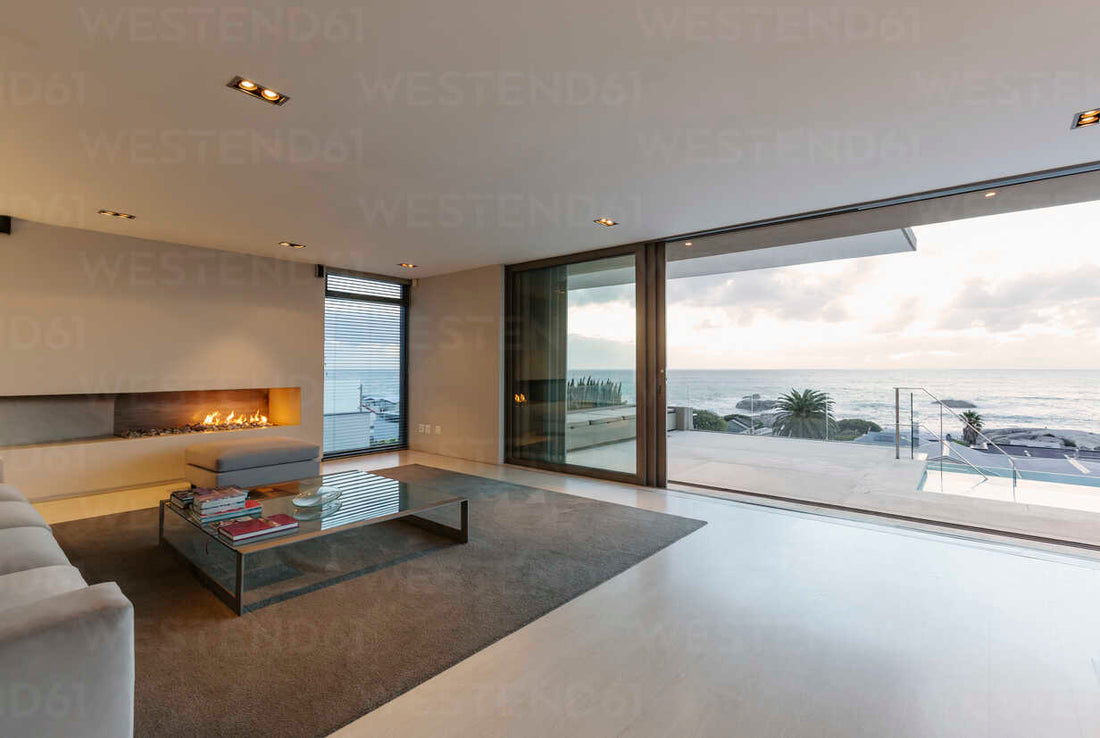This image captures the interior of a modern living room with a stunning ocean view. The room features expansive glass patio doors stretching from one side to the other, seamlessly connecting the cozy indoor space to a cement patio outside. Beyond the patio, a few steps lead down to a glistening swimming pool, all framed by the serene backdrop of the ocean and a bright sky peppered with clouds. 

Inside, the living room is characterized by an off-white color palette, with a creamy ceiling adorned with track lighting and white tile flooring. An off-white sofa, adorned with four light cushions, sits prominently on a large, dark brown throw rug that occupies much of the floor space. There's a matching footstool beside the sofa, complementing the room's cohesive look. 

At the center of the rug stands a rectangular glass coffee table with pewter-colored metal trim, displaying a few books and a knick-knack. To the left, a beige wall features a sleek, built-in fireplace with a narrow horizontal slit extending across the wall, where vibrant orange flames dance, casting a warm glow. Adjacent to the fireplace, a window offers an additional glimpse of the ocean view, maximizing the room's connection to the stunning seascape outside.

The ceiling is dotted with rectangular indentations housing double light bulbs, contributing to the room's modern aesthetic. Moreover, the bottom right corner showcases the pristine white cream flooring, reinforcing the room's bright and airy atmosphere. Finally, it's notable that the image is watermarked with "WESTEND61" throughout, indicating its source.